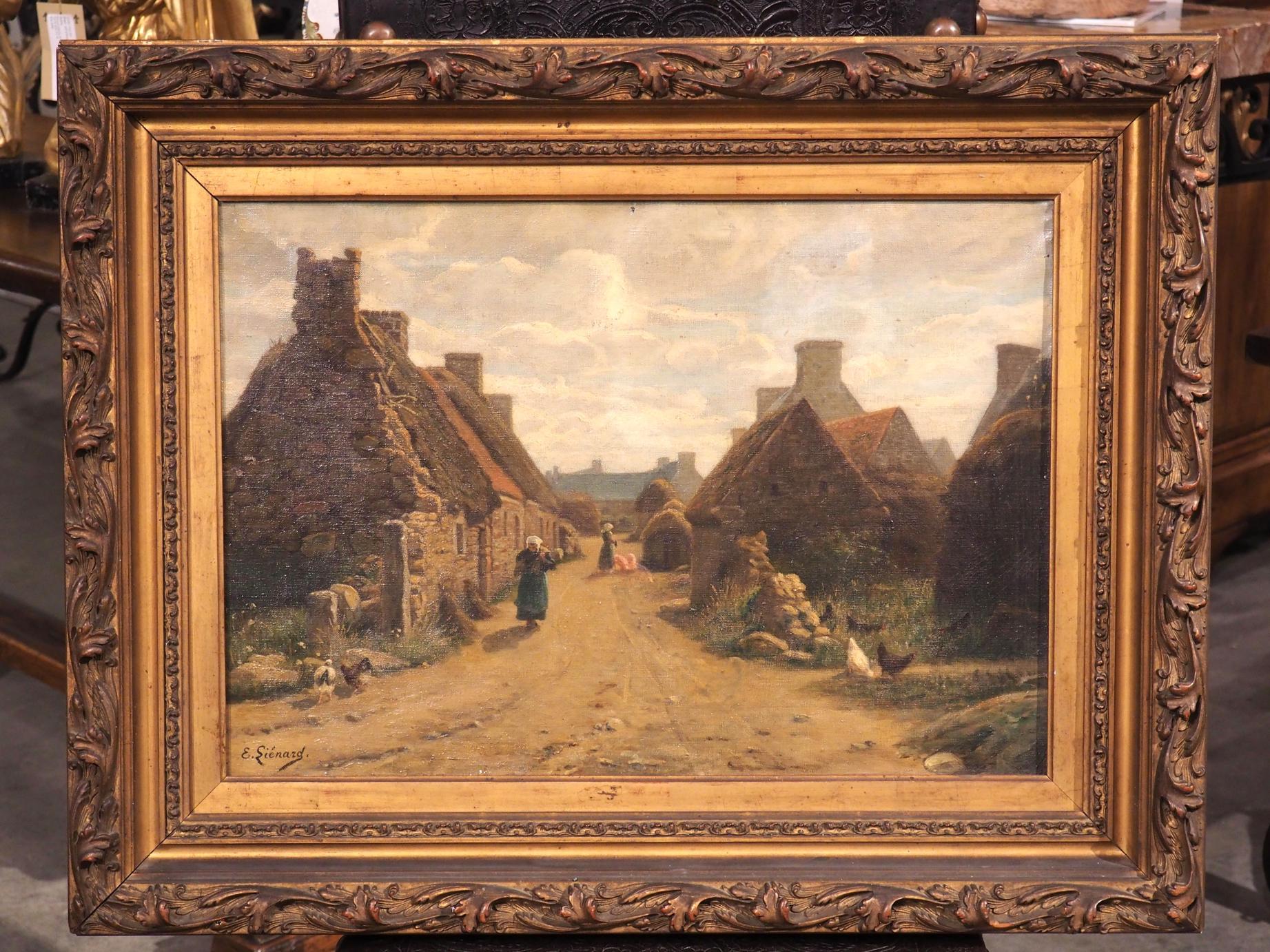The image depicts an antique, intricately detailed painting housed in an ornate, hand-carved wooden frame featuring a decorative leaf and scroll design. The painting itself is horizontal and further encased within several inner frames, including a gold-toned one. The scene captures a medieval village characterized by a central light brown dirt road that bisects the town. To the left, stand robust homes with stone walls, large fireplace chimneys, and red triangular wooden roofs. To the right, there are smaller, similarly built homes. In the background, the structures transition into even smaller huts with grass roofs.

Along the dirt path that leads into the distance, green patches of weeds flourish at the forefront, while roosters and chickens amble about. Women clad in long dresses and white head coverings are also visible, contributing to the lively medieval atmosphere. Overhead, the sky is an evocative blend of wispy orange, blue, and white hues, complementing the old-world charm of the oil painting.